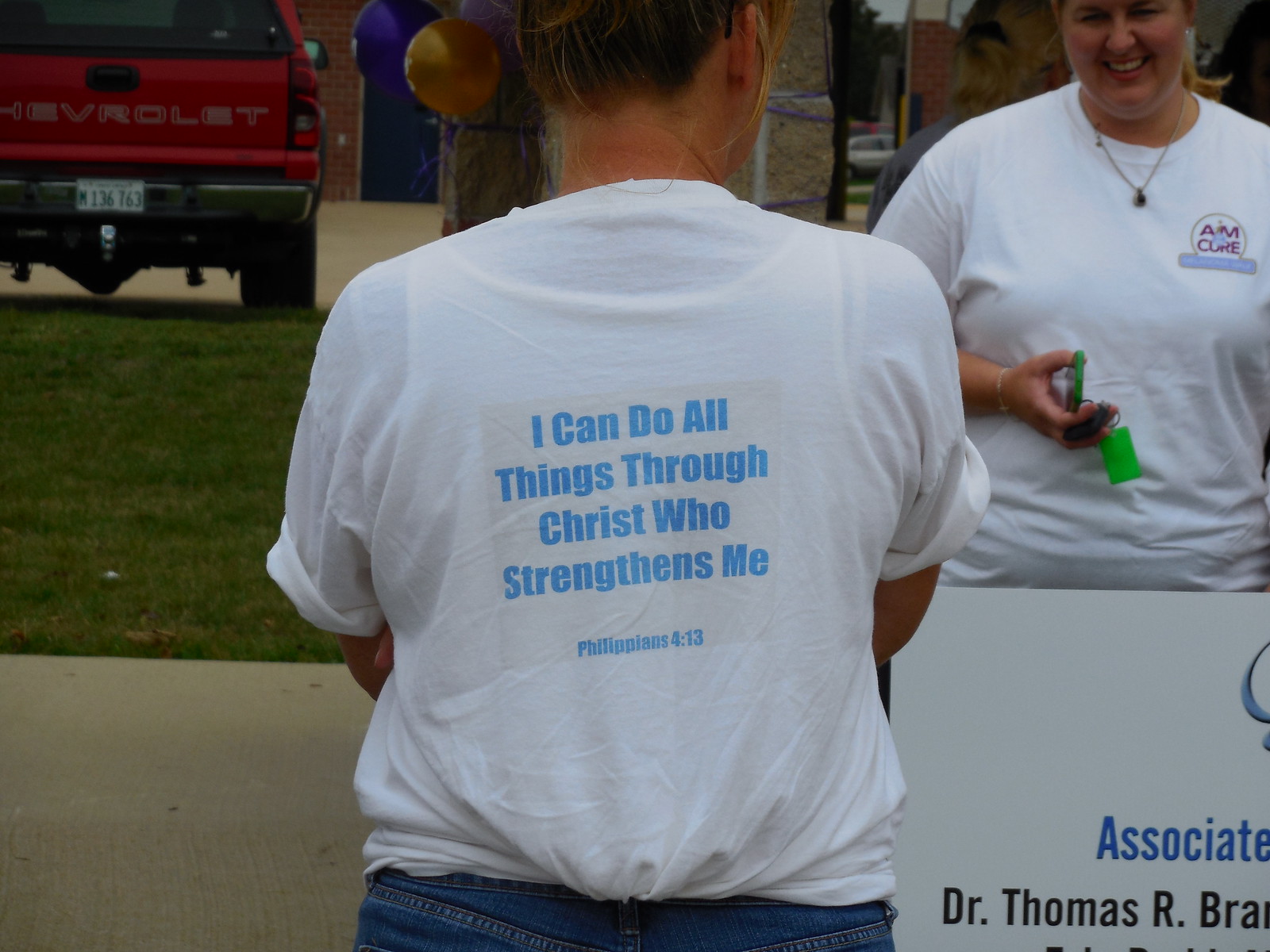The image captures an outdoor scene featuring two individuals positioned around a sign. In the center of the frame is a man with his back to the camera, wearing a white t-shirt and blue jeans. The back of his shirt prominently displays a blue-printed Biblical quote, "I can do all things through Christ who strengthens me. Philippians 4:13." To his right stands a smiling woman, partially obscured by a white poster that reads "associate Dr. Thomas RAB..."—the rest of the text cut off by the frame's edge. She wears a white t-shirt with "a.m. Core" printed on it and holds a green key fob in her hand. The woman appears to be in her late 30s and has a slightly overweight build. The scene is set outdoors with a grassy yard to the left, a red Chevrolet pickup truck parked nearby, a brick building in the background, and a column adorned with blue and gold balloons. Their attire, along with the textual references, suggests a Christian association gathering.